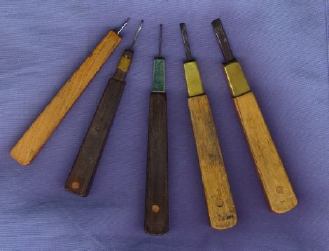This is an overhead photograph featuring five handheld artist tools for oil painting, arranged in an arch on a purple surface. All five tools have wooden handles, with three showcasing a worn, light tan color, and two exhibiting a darker brown hue. The brass fittings on the handles indicate their connection to the metal implements, which differ in shape and size. Among the tools, three have slender, pointed ends, resembling needles, while the other two are broader and flatter. The metal ends appear old and well-used, characterized by a rusty patina. The arrangement and condition of these tools suggest they have been essential instruments in various artistic endeavors.